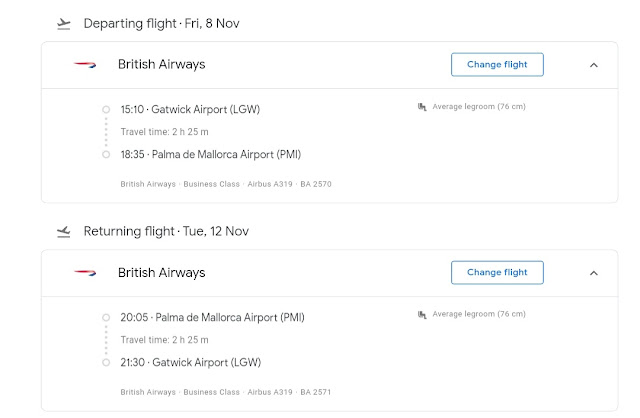A detailed flight schedule is displayed on a clean white page. At the top left, the grey text reads "Departing Flight Friday 8th November" with a small grey icon of a plane taking off positioned beside it. Below this header, in a highlighted box, "British Airways" is prominently displayed next to a red and blue logo. Adjacent to this, there's a button labeled "Change Flight."

Further down, the schedule shows: 
- Departure at 05:10 from Gatwick Airport (LGW), 
- An annotation "Average Living Room 76cm,"
- A travel duration of 2 hours and 25 minutes,
- Arrival at 18:35 at Palma de Mallorca Airport (PMI).

Additional information includes "British Airways Business Class Airbus A319 BA2570" written in grey text. 

The schedule also details the return flight:
- "Returning Flight Tuesday 12th November" in a similar format.
- "British Airways" is displayed again, 
- Departure at 20:05 from Palma de Mallorca Airport (PMI),
- Travel time listed as 2 hours and 25 minutes,
- Arrival at 21:30 at Gatwick Airport (LGW), with the same aircraft details and class listed: "British Airways Business Class Airbus A319 BA2570" in grey text.